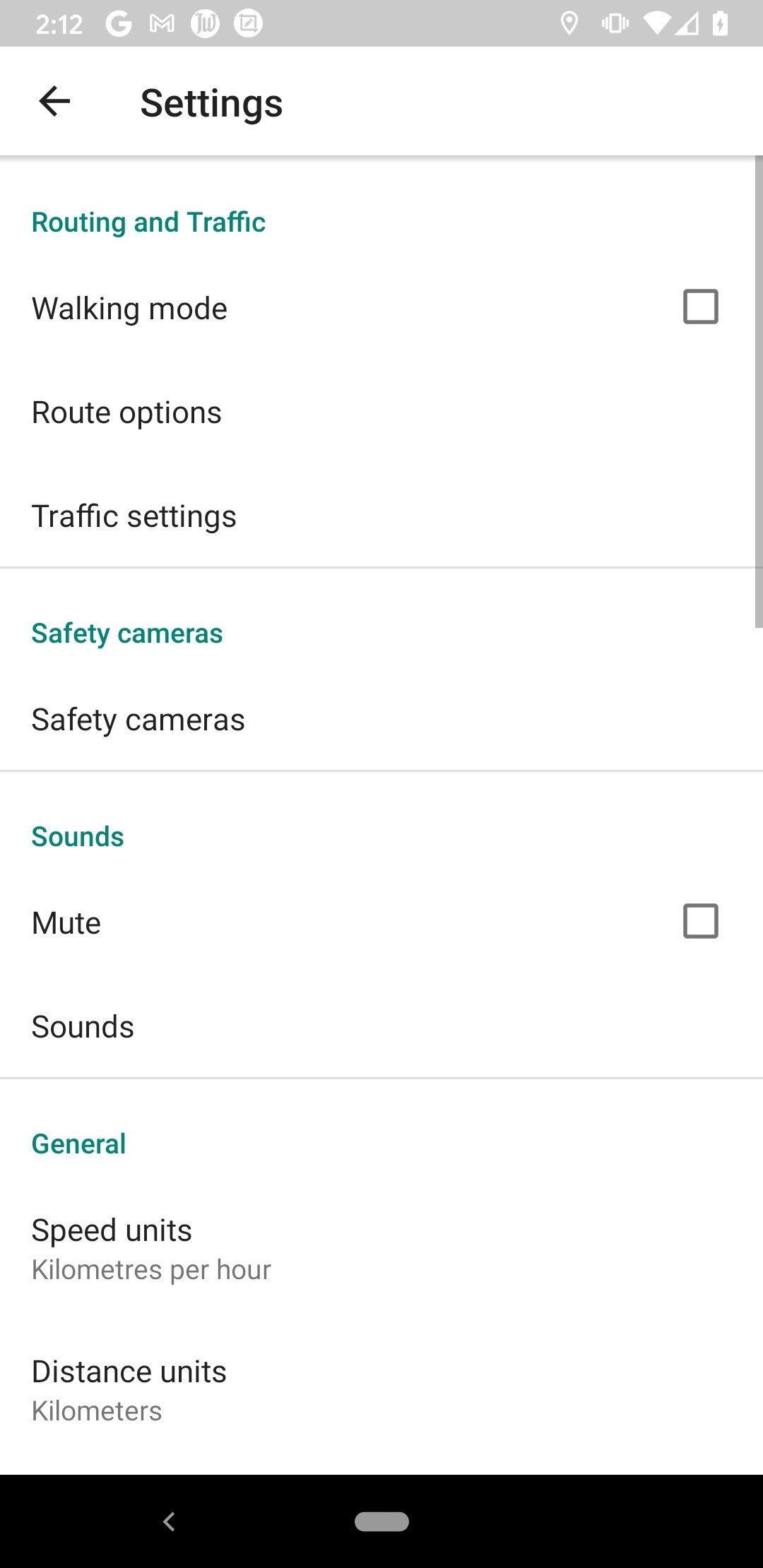The image is a screenshot from a cell phone, featuring a comprehensive view of various interface elements and settings. At the very top, a gray status bar displays several indicators from left to right: the number '212', followed by icons for Google, Gmail, 'JW', location, vibrate mode, Wi-Fi, and battery.

Below the status bar, there is a black arrow pointing to the left next to the word 'Settings' indicating a navigation option. The screen subsequently lists multiple menu items in a vertical layout: 'Routing and traffic', 'Walking mode', 'Route options', 'Traffic settings', 'Safety cameras' (appearing twice), 'Sounds', 'Mute', 'Sounds' again, 'General', 'Speed units' labeled as 'Kilometers per hour', and 'Distance units' labeled as 'Kilometers'.

At the bottom of the screen, a black border spans horizontally, containing a white left-pointing arrow and a gray oblong shape in the center, possibly representing a navigation or selection button. The screenshot is devoid of any photographic elements, people, animals, plants, flowers, or trees. The image has a vertical orientation, being taller than it is wide.